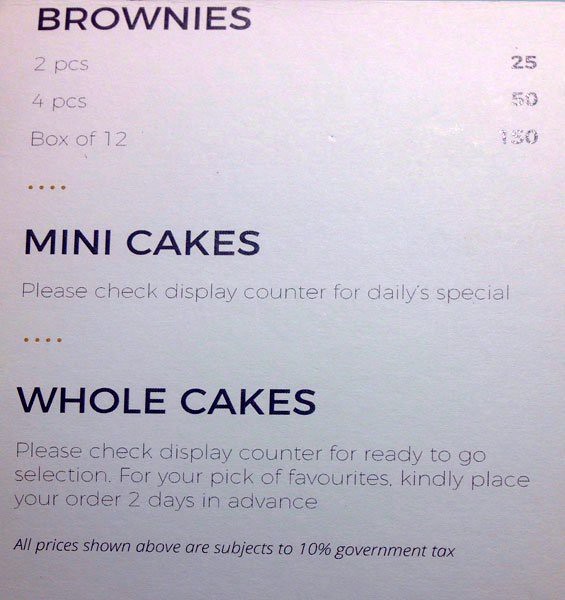This photograph features a detailed white paper menu listing three types of items: brownies, mini cakes, and whole cakes. At the top, in bold capital letters, the menu item "BROWNIES" is displayed, followed by pricing in smaller letters: Two pieces, 25; Four pieces, 50; Box of 12, 150. Below this, separated by a subtle visual divider, "MINI CAKES" is written in bold capital letters, instructing customers to "Please check display counter for daily special." Following another divider, "WHOLE CAKES" is also in bold capital letters, with a note beneath: "Please check display counter for ready to go selection. For your pick of favourites, kindly place your order 2 days in advance." At the bottom of the menu, there's a disclaimer stating that "All prices shown above are subject to 10% government tax."